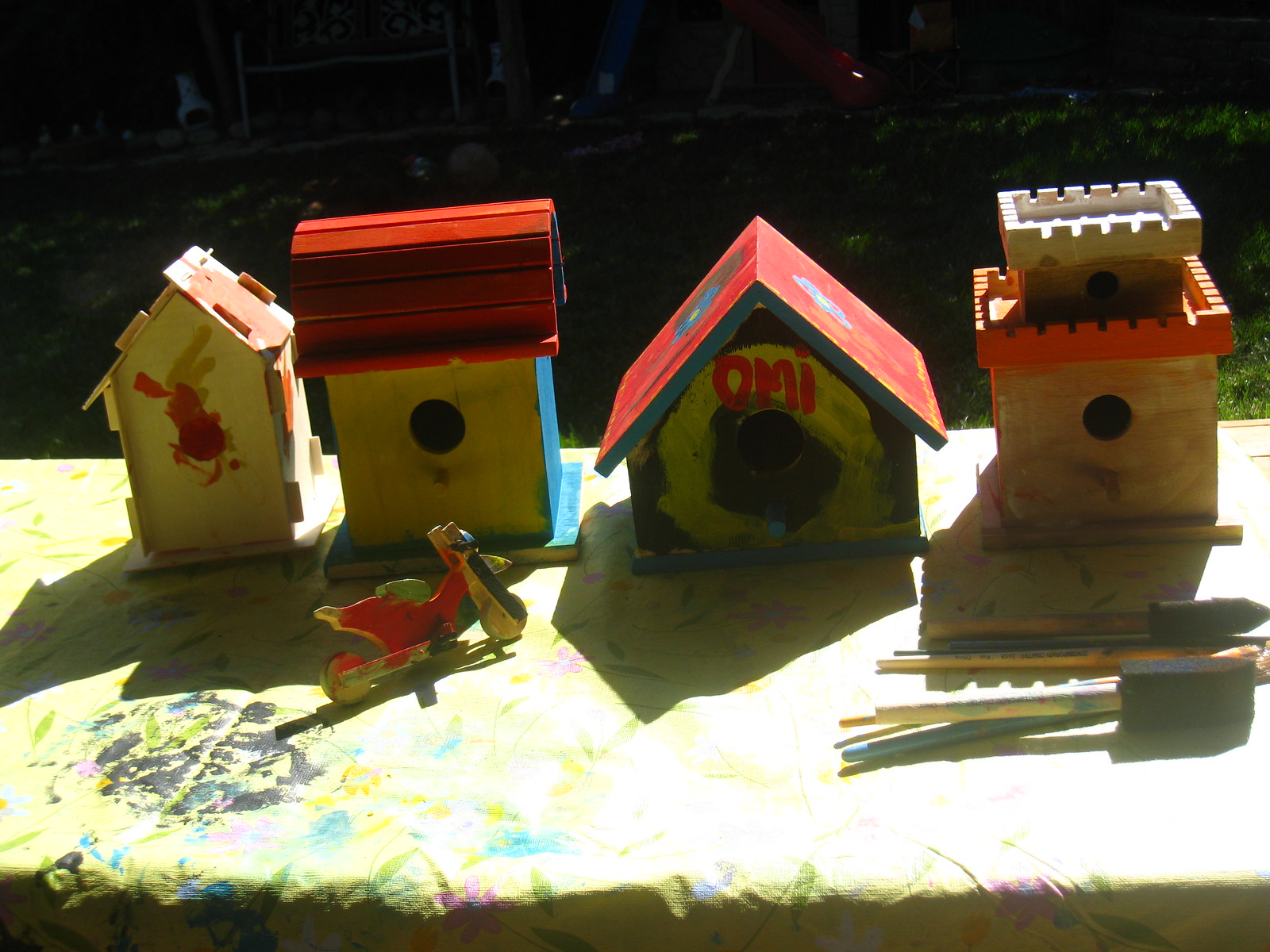The photograph showcases four homemade, wooden birdhouses arranged on a yellow-green table, reminiscent of a child's table. Surrounding the birdhouses are assorted paintbrushes and sponges, suggesting that the painting was part of a children's crafting project. The table itself is set against a dark background, possibly illuminated by moonlight or a streetlamp, enhancing the focus on the birdhouses. Each birdhouse features a small circular opening and is painted with various colors—black, red, yellow, beige, and blue—in a messy, unrefined manner typical of children's artwork. Notably, one birdhouse bears the name "Amy." In addition to the birdhouses, there's a partially painted wooden bicycle or motorcycle on the table, sharing the same color palette. These handcrafted items, likely intended for use in a garden, rest on a paint-stained drop cloth, highlighting the creative and playful nature of the project.